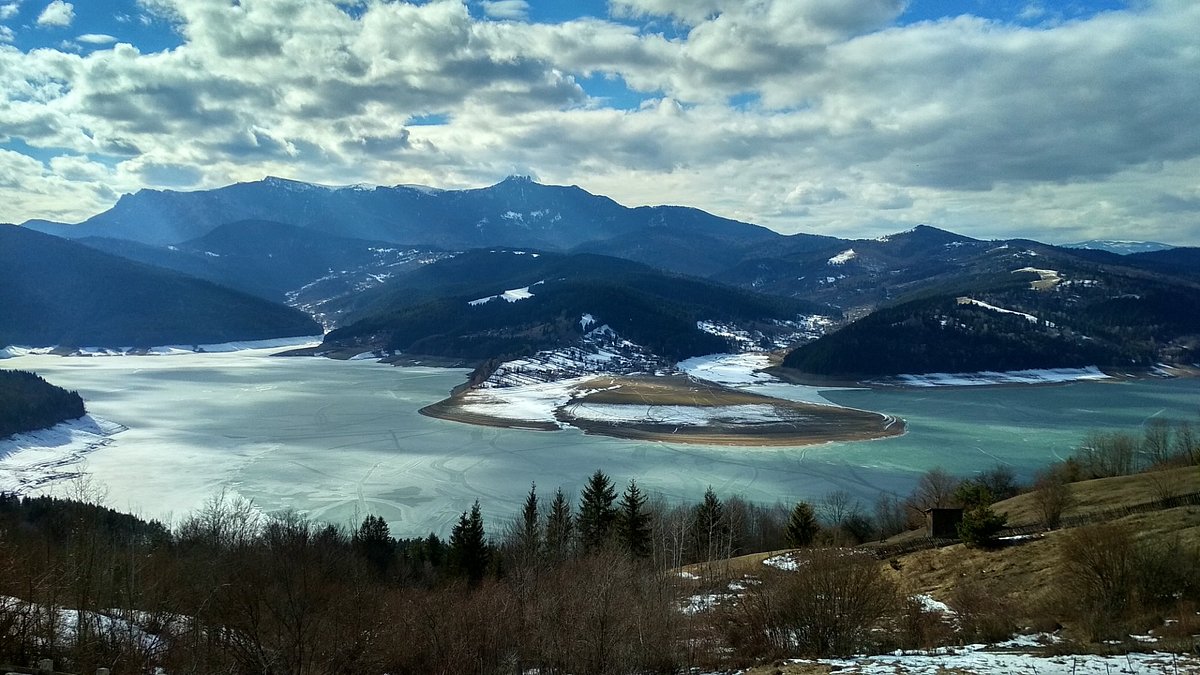This detailed landscape photograph captures a serene winter scene from the top of a tall hill or mountain. The perspective offers a sweeping view over a partially frozen lake or river, flanked by tree-lined slopes. Both evergreen and deciduous trees populate the foreground, the latter with bare branches indicative of the season. Snow patches dot the brownish-green ground and the trees, emphasizing the wintry atmosphere. Central to the image is a brownish landmass covered in dead grass and snow, seemingly rising toward a mountainous range in the background. The distant mountains exhibit scattered snow patches and snow-capped peaks, with some buildings faintly visible on one of the slopes. The sky above is a mixture of blue and white, with a blend of clouds allowing hints of blue to peek through, contributing to the tranquil, cold aesthetic of the scene.